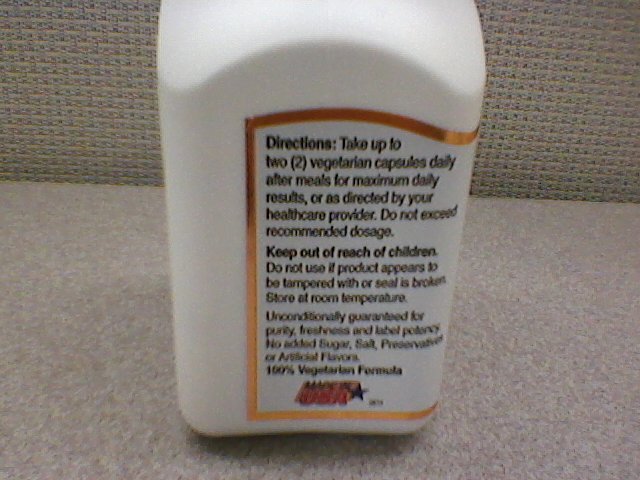Caption: 

An opaque white bottle is prominently displayed within a room. The side of the bottle presented in the image features a white label with a shiny orange border and black text. The label provides detailed usage instructions, advising the consumption of up to two vegetarian capsules daily after meals for optimal results, or as per a healthcare provider's guidance. It stresses not to exceed the recommended dosage and to keep the product out of children's reach. The text also warns against using the bottle if it appears tampered with or if the seals are broken. The bottle should be stored at room temperature. The label emphasizes the product’s purity, freshness, and adherence to label guarantees, noting that it contains no additional sugar, salt, preservatives, or artificial flavors.